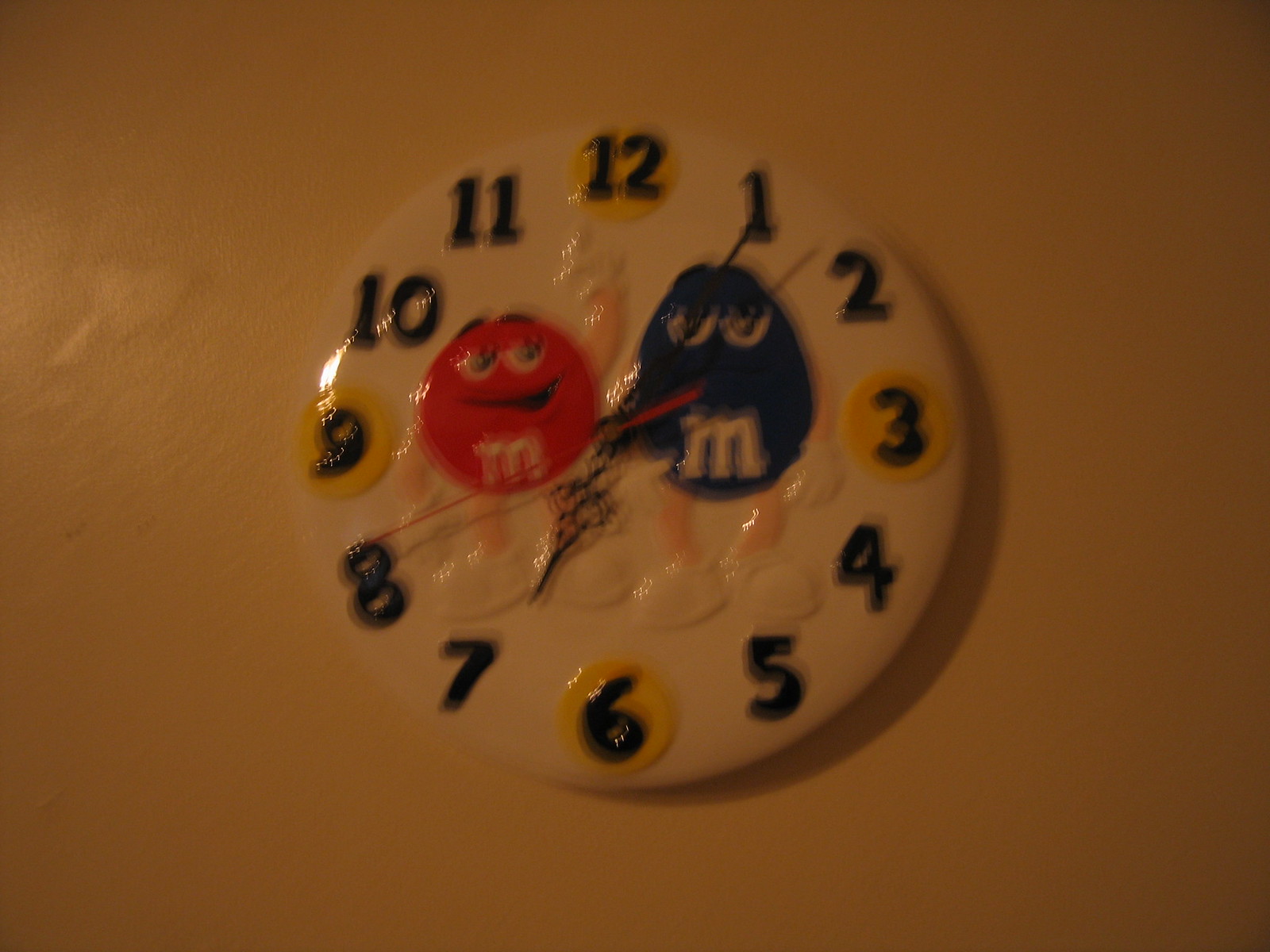The image showcases a light brown, beige wallpaper serving as a backdrop for a whimsical M&M-themed clock. The clock face is adorned with circles mimicking M&Ms, colored in blue and yellow representing the numbers 1 through 12. Particularly, the 12, 3, 6, and 9 positions are highlighted with larger yellow circles. The hour and minute hands are crafted from black metal, while the second hand is conspicuously red. The clock displays the time at 6:05. At the center of the clock, there are two M&M characters: a larger blue peanut M&M with arms resting at its sides, and a smaller red M&M with one arm animatedly pointing upward. This playful centerpiece adds a delightful touch to the otherwise simple clock design.